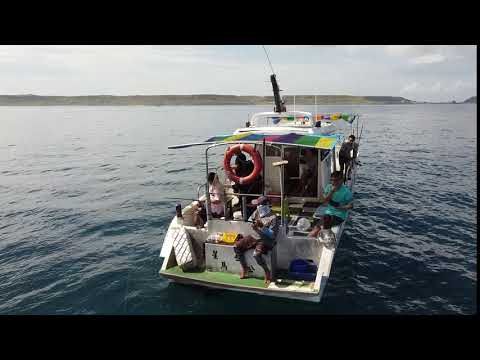In the image, a small boat floats on a large body of calm, blue water, which could either be an ocean or a lake. The boat bears a striking resemblance to the one from the movie "Jaws," minus an upper deck where the person drives. Instead, the cockpit is located inside the cabin. Above the boat, the sky is filled with white clouds, and in the distant background, there is a rocky or mountainous landscape that appears gray.

The boat itself is white with a rainbow-colored canopy stretching across its top, featuring stripes that go from yellow to green, purple, pink, blue, and then yellow again. A red and white life preserver is prominently displayed on the back, where a man, possibly wearing camouflage clothing, is seated beneath it. Nearby, a woman in a dress is perched on the edge of the boat, watched over by another man positioned in front of her.

There are about six or seven people onboard, appearing to be of either Asian or African-American descent. All passengers seem to have covers over their mouths, and their clothing varies from lighter colors to blue shirts and gray shorts, along with vivid accents like reddish pants. Despite the boat's small size that leaves the passengers somewhat cramped, they seem to be enjoying either a fishing trip or leisure time. The boat also features a shaded booth area at the back, completing the overall scene of a packed yet pleasant outing on a serene water body.